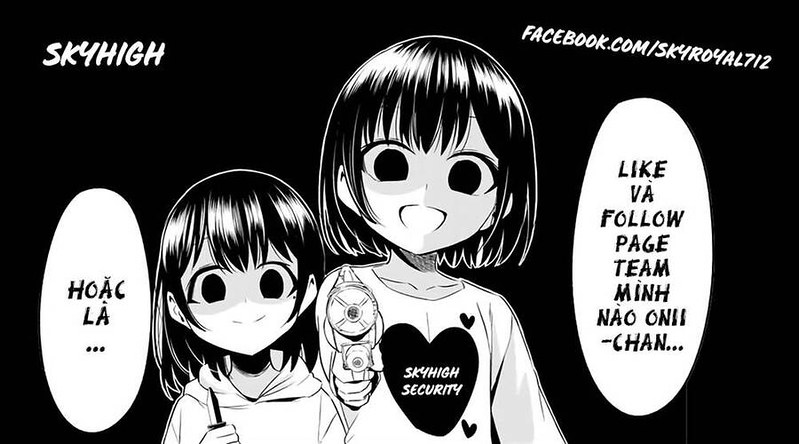The image is a meme taken from a famous Japanese manga, rendered in a distinctive black and white anime style. It features two young girls with exaggerated facial expressions and big eyes, standing out against a stark black background. In the upper left corner, white text reads "Sky High," while the upper right corner displays the text "Facebook.com/SkyRoyal712."

On the left side of the image, a shorter girl with shoulder-length black hair and a big smile is depicted. She is wearing a white hoodie and holding a knife. Next to her in a speech bubble with black text, it reads "H-O-A-C-L-A..."

On the right, a slightly taller girl with similar shoulder-length black hair, also smiling broadly, is shown. She is wearing a white shirt branded "Sky High Security" with a heart symbol and is holding a gun. To the right of her, in a larger speech bubble, white text reads "Like VA Follow Page Team M-I-N-H-N-A-O-O-N-I-I-C-H-A-N." The image’s contrasting black background accentuates the white text and the expressive characters, giving the scene a dramatic and eye-catching appeal.